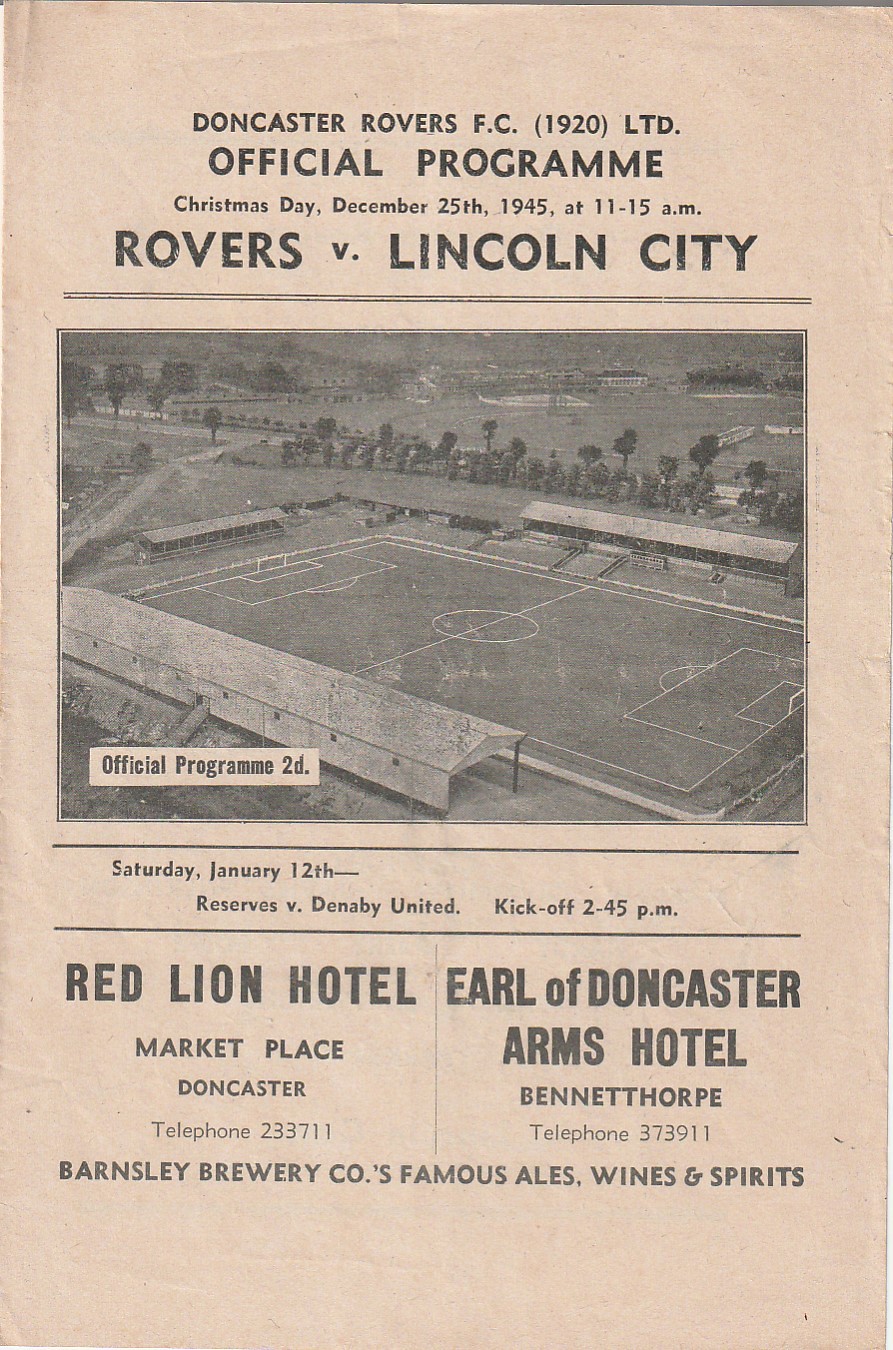This detailed image captures the scan of an aged, crinkled program booklet from a 1945 football (soccer) match. The formerly white paper has aged to a light tan or gray hue, giving it a vintage feel. Centrally positioned, a black and white photograph depicts a soccer pitch, framed by a surrounding row of trees and fields in the background.

At the very top, bold letters announce "Doncaster Rovers FC (1920) LTD Official Program", specifically for the Christmas Day match on December 25th, 1945, at 11:15 a.m., featuring "Rovers vs. Lincoln City". Adding authenticity and historical context, the program includes details of a subsequent reserve match: "Saturday, January 12th, Reserves v. Denbigh United, kickoff, 2:45 p.m." This is underlined, separating it from the ads below.

The lower half of the program prominently displays sponsor advertisements. On the left, it reads "Red Lion Hotel, Marketplace, Doncaster, telephone: 233711" and on the right, "Earl of Doncaster Arms Hotel, Bennetthorpe, telephone: 373911". Beneath these, in a smaller font, is an ad for "Barnsley Brewery Company's Famous Ales, Wines, and Spirits."

The aged cream and black tones contribute to the nostalgic essence, while the meticulous text placement enhances the historical significance of this football program.